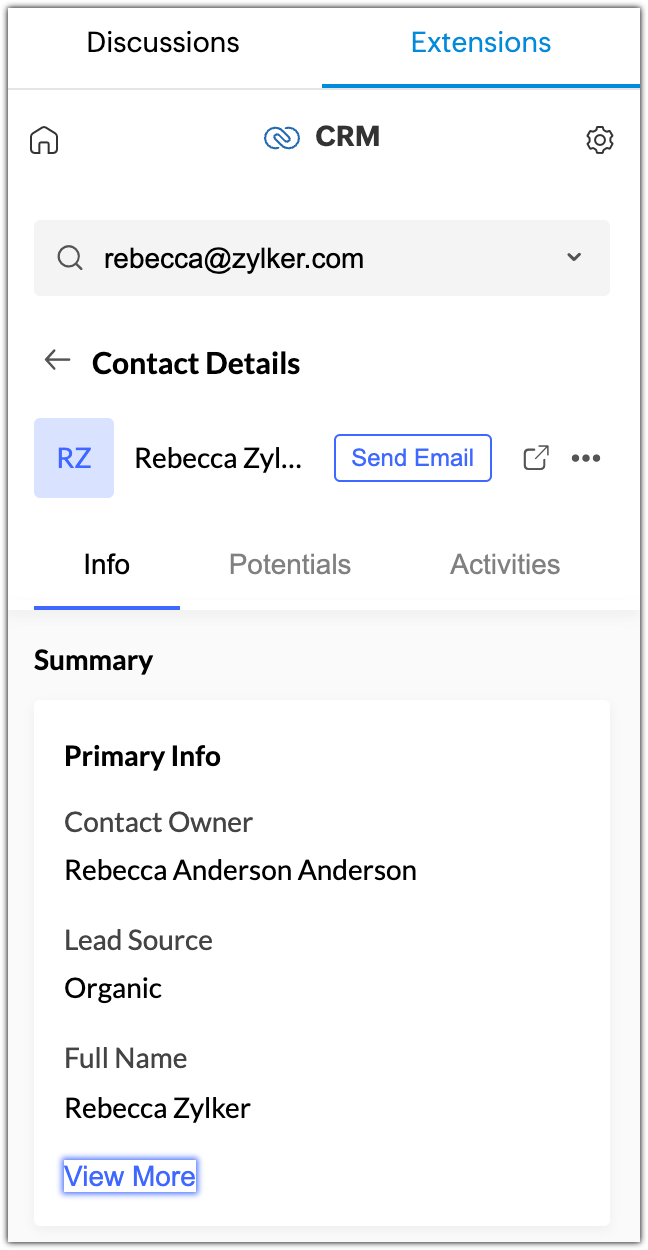The image displays a detailed page within a CRM platform, highlighting various sections and elements. At the top of the page, there are tabs labeled "Discussions" and "Extensions," with "Extensions" emphasized in blue text and underlined with a blue line.

Directly below this, there is a navigation bar featuring a home icon on the left, a chain link icon with "CRM" in the middle, and a gear icon on the right. Underneath this bar, there is a search magnifying glass icon accompanied by "Rebecca@Zylker.com," along with a dropdown menu denoted by an arrow to the right of the email.

Further down, a back arrow is followed by the bold heading "Contact Details." Next to this heading, there is a blue square with the initials "RZ" on it, indicating part of the user's name: "Rebecca, Z-Y-L..." Next to this is a simple button with "Send Email" in blue text on a white background, which also includes a blue horizontal line and a pop-out area to the right of it.

Below this section, there are three tabs labeled "Info," "Potentials," and "Activities." "Info" is in black text with a blue underline, indicating it is the current selection, while "Potentials" and "Activities" are in gray text.

Under the "Info" tab, there is a bold subheading labeled "Summary" followed by an indented, bold section titled "Primary Info." Details within this section include "Contact Owner: Rebecca Anderson Anderson," "Lead Source: Organic," and "Full Name: Rebecca Zylker." At the very bottom of the section, there is a "View More" button.

This comprehensive layout organizes crucial CRM information efficiently, presenting navigation links, contact details, and primary information in a user-friendly and visually structured manner.